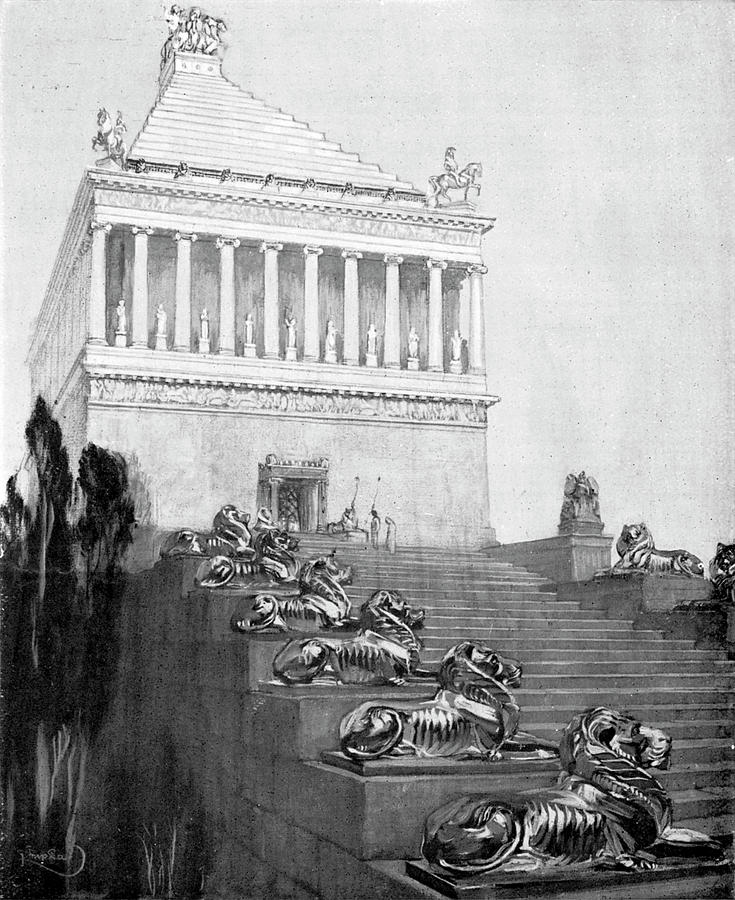This intricate black-and-white illustration, in portrait orientation, depicts an imposing ancient-style temple that combines elements of Greek and Roman architecture. The temple is perched atop a grand set of stone stairs, which are flanked by a series of meticulously sculpted, resting lion statues that collectively face inward towards the stairway. The structure itself is predominantly stone and stands two stories tall with a stepped pyramid, or ziggurat-like, roof. At the corners of this roof, there are statues of horses rearing up with riders astride them, accentuating the grandeur. The frontage of the temple is marked by an array of white pillars, topped and bottomed with ornate filigree details, and interspersed with additional smaller statues or figurines on pedestals. The entrance on the ground floor is a single, prominent door between two pillars, leading the eye upwards towards the more elaborately adorned second floor. Sparse shrubs are visible on the far left side, adding a touch of nature to an otherwise austere scene devoid of other discernible foreground or background features.